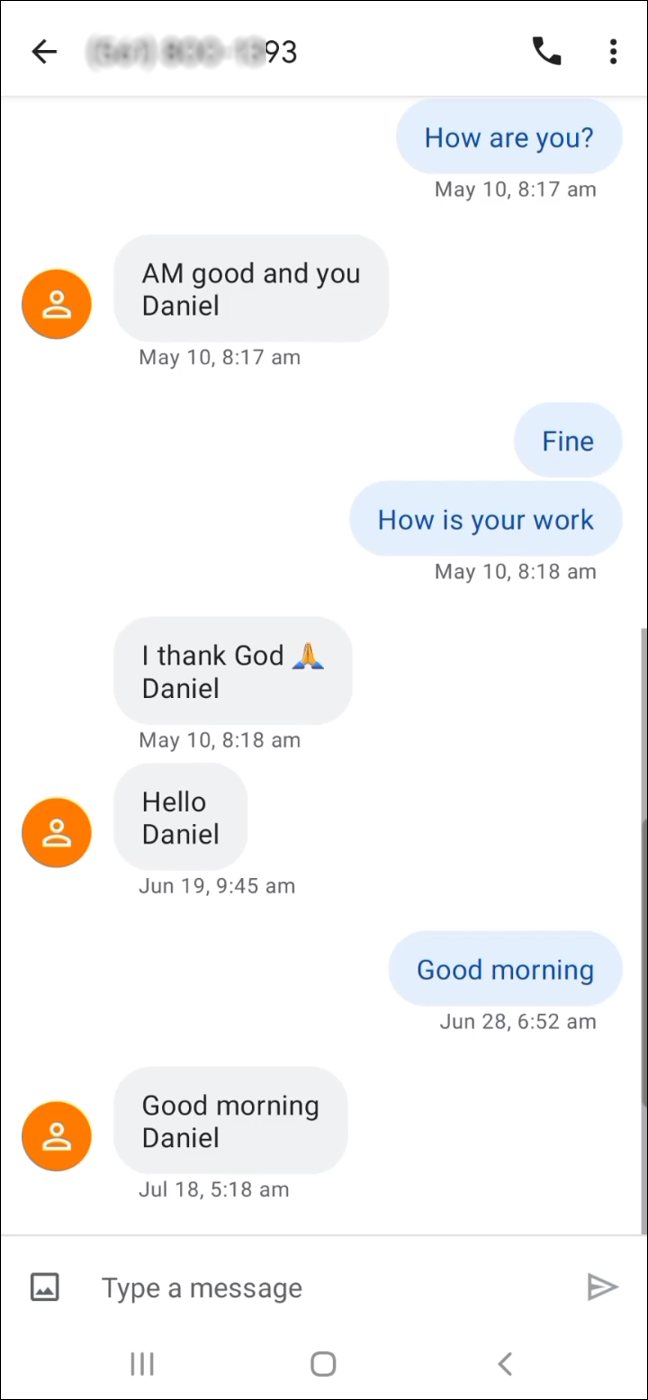The screenshot captures a snippet of a conversation on a messaging app, marked by various user interface elements. 

At the top of the screen, there is a navigation arrow pointing to the left, rendered in black. Beside it, a phone number appears, but it has been obscured for privacy. Adjacent to the phone number are a phone icon and a menu represented by three vertical dots.

The chat window below showcases an exchange between two individuals, represented by blue and light gray message bubbles. The conversation unfolds as follows:

1. Blue Bubble: "How are you?"
2. Light Gray Bubble: "Am good, and you, Daniel?"
3. Blue Bubble: "Fine, how is your work?"
4. Light Gray Bubble: "I thank God, Daniel 🙏"

The dialogue continues with:
1. Light Gray Bubble: "Hello, Daniel."
2. Blue Bubble: "Good morning."
3. Light Gray Bubble: "Good morning, Daniel."

Below this last exchange, there is a horizontal line, under which lies a small square icon depicting mountains—likely indicating the option to add a photo. At the very bottom, there is a text input field labeled "Type a message," accompanied by a send arrow pointing to the right.

Overall, the screenshot effectively captures a typical, cordial conversation between two individuals on a messaging platform, providing insight into the app's structural and visual layout.